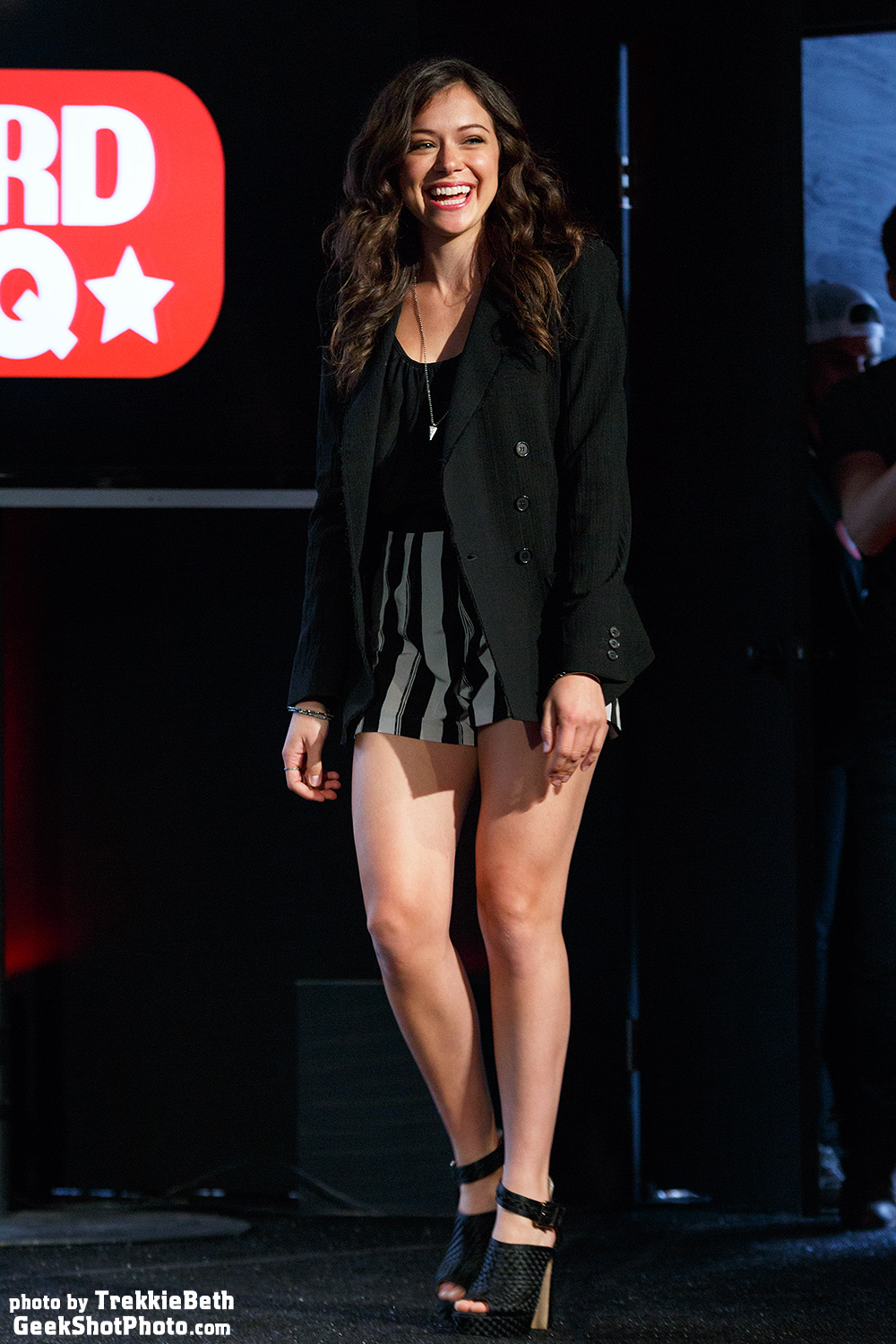In this digital photograph, a young woman, possibly of Latino descent, stands center stage in what appears to be an indoor venue, potentially a talk show studio or nightclub. She has long, dark, curly hair styled in waves, possibly with a curling iron. The woman is captured laughing and smiling widely, looking slightly off to the right. She is dressed in a chic ensemble consisting of a black tank top under a black blazer jacket, paired with black and gray or black and white short shorts, which end well above her knees. Her accessories include a long silver chain necklace and two bracelets, and she completes her outfit with black high-heeled shoes.

In the background, there are signs and a couple of other people, indicating a lively atmosphere. A prominent red sign with white letters and a star is situated to the left of the image. The carpeted floor and other elements, such as people and additional signage, suggest the setting is indoors. The bottom left-hand corner of the photograph contains the text "Photo by Trekkie Beth, GeekShotPhoto.com." The overall color palette includes red, white, black, gray, tan, and pink.